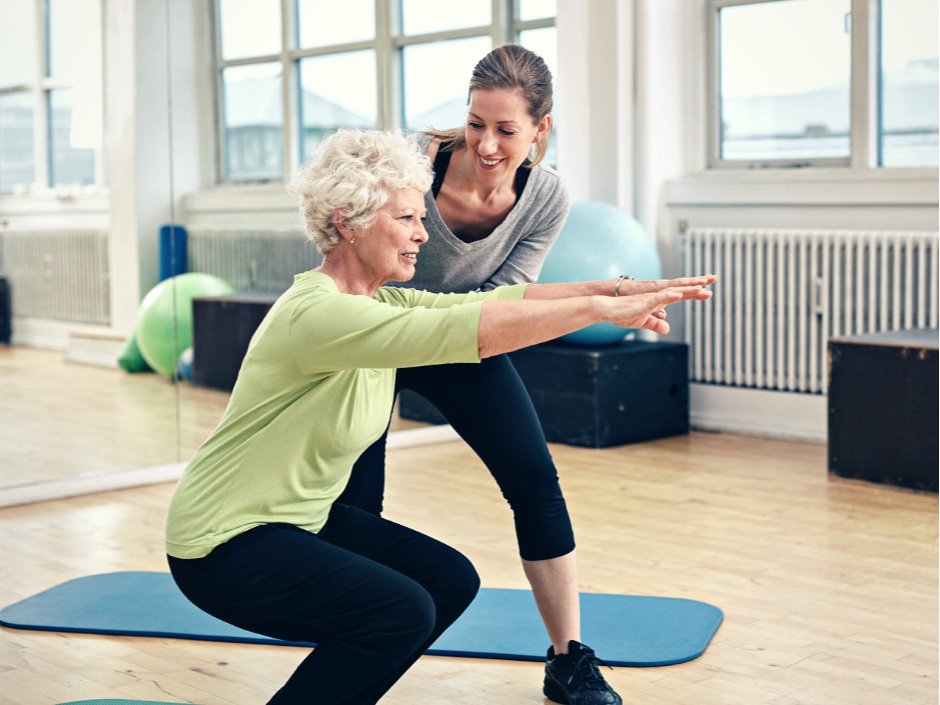In a serene, light-filled yoga studio with white walls and large windows, an older woman with short white hair is engaged in a yoga pose, extending her arms in front of her. She wears a soft pale green shirt with three-quarter length sleeves and black yoga pants, standing on a light blue yoga mat that spans from the left corner towards the center right of the room. The instructor, a younger woman with dark hair pulled back into a ponytail, stands close by, providing support and guidance with a warm smile. The instructor is dressed in a gray shirt over a black tank top, black leggings, and black shoes. The studio features light wooden hardwood floors, a white painted radiator in the upper right corner, and a wall of windows that offer a view of other buildings. Various exercise equipment, including black wooden trunks, a large light blue yoga ball, and a green exercise ball reflected in a wall-length mirror, are neatly arranged along the walls, adding to the organized and peaceful ambiance of the space.